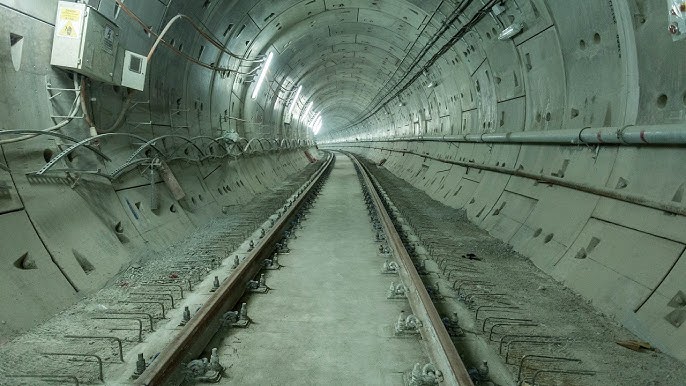This detailed, full-color photograph depicts a long, underground tunnel with a circular, rounded structure and a flat floor. The tunnel, likely part of an underground facility, is illuminated by artificial lighting that is focused on the upper center and along the left side, though overall the scene appears in shades of gray with a slightly greenish hue. Stretching deep into the distance, the tunnel curves gently to the left and is lined with numerous small, bent metal pieces protruding from both sides, which may serve structural or functional purposes. Along the sides of the tunnel, there are pipes or tubing, suggesting the presence of utility lines, including possible wires for power or oxygen supply. On the top left, a power or electrical box is mounted. The floor features rails reminiscent of train tracks, suggesting a railway system used to transport people or materials within the facility. Despite the sparse lighting fixtures, the tunnel remains brightly lit, highlighting its meticulous and streamlined construction.